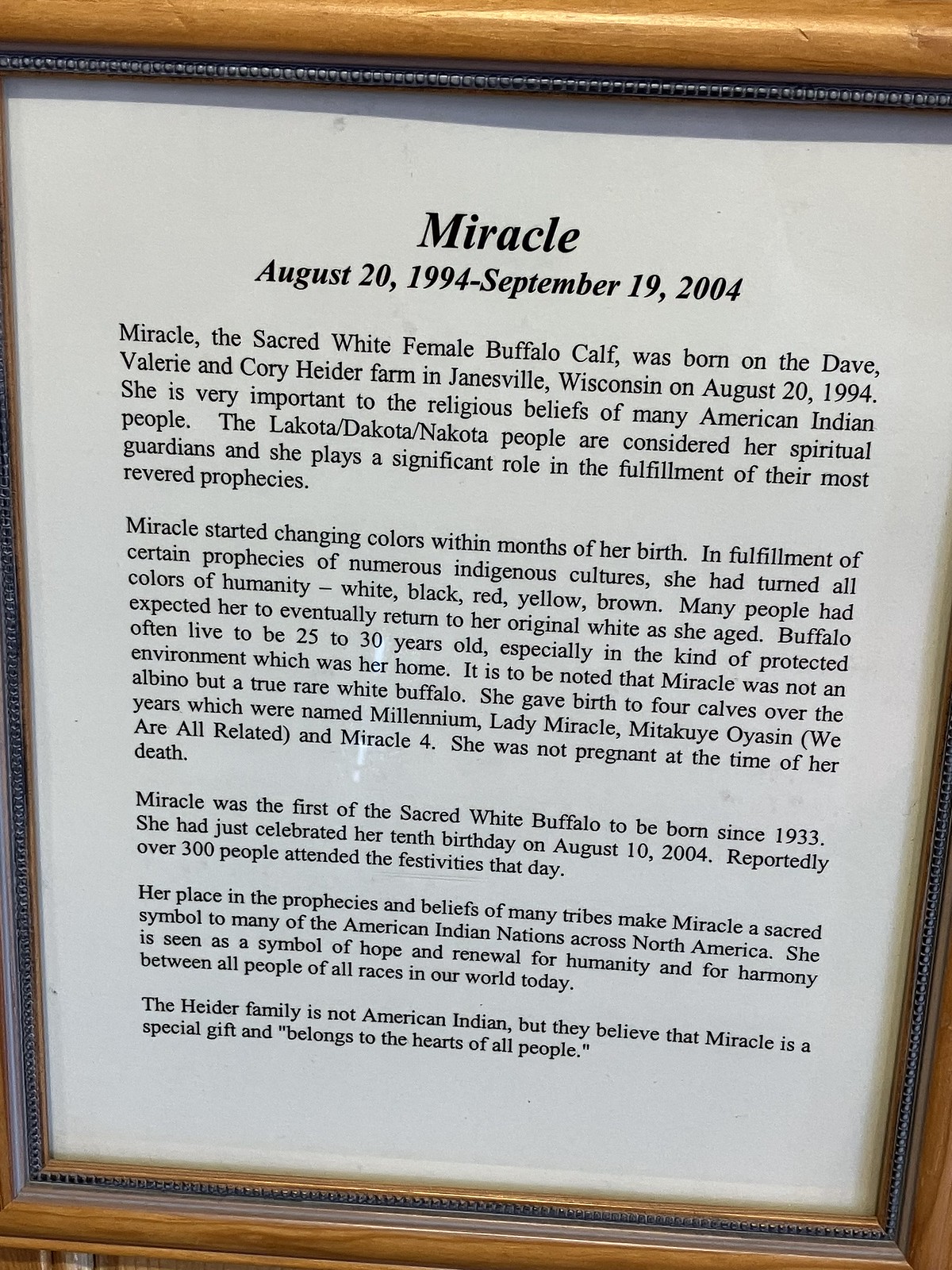This photograph captures a framed, vertically-oriented commemoration article, surrounded by a brown and yellow wooden border. The white background holds black typed text detailing the significance of Miracle, the sacred white female buffalo calf. At the top center, bold letters proclaim "Miracle," followed by her lifespan, "August 20, 1994 to September 19, 2004." 

Miracle was born on the Dave, Valerie, and Corey Heider farm in Janesville, Wisconsin, and holds great importance to the religious beliefs of many American Indian tribes, particularly the Lakota, Dakota, and Nakota peoples who are considered her spiritual guardians. She began to change colors within months of her birth, turning shades of white, black, red, yellow, and brown, thus fulfilling various indigenous prophecies. Though expected to return to her original white as she aged, Miracle remained a symbolic figure of hope and renewal for harmony among all races.

The article notes that Miracle was not an albino but a true rare white buffalo. She gave birth to four calves named Millennium, Lady Miracle, Mitakuy Oyasin (meaning "we are all related"), and Miracle Four. Though typically buffalo can live up to 30 years in protected environments, Miracle passed away shortly after her 10th birthday, which had been celebrated by over 300 attendees on August 20, 2004. She holds a sacred place in the prophecies and beliefs of many tribes across North America, regarded as a sacred symbol with a significant spiritual impact. Despite not being of American Indian descent, the Heider family revered Miracle as a special gift belonging to all hearts.